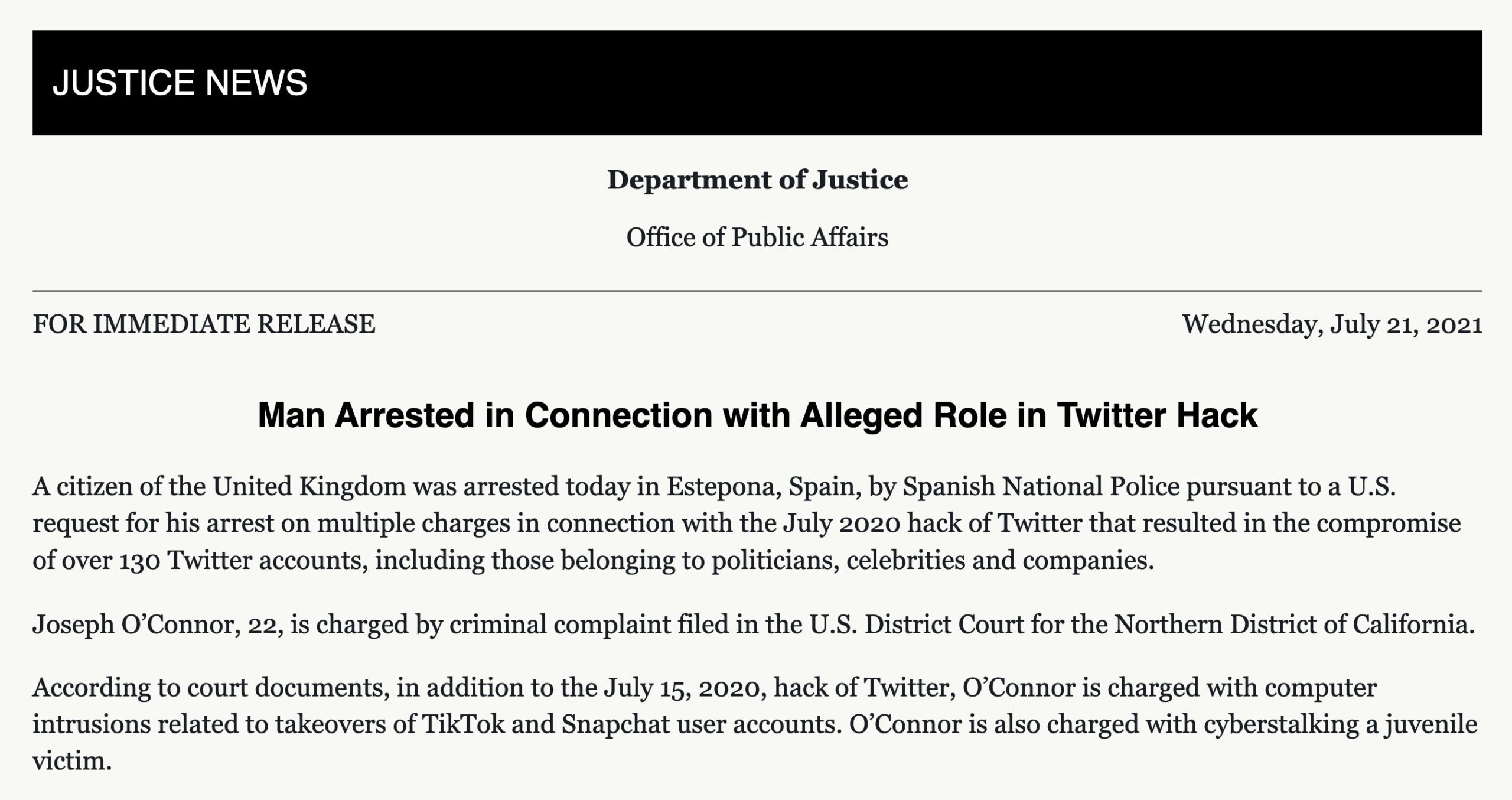In the top left corner of the banner, "Justice News" is displayed in black text on a white background. Below this, the text reads "Department of Justice," followed by "Office of Public Affairs." A green line runs beneath these titles. On the left side, the text reads "For Immediate Release," and on the right, "Wednesday, July 21, 2021."

The main headline states: "Man Arrested in Connection with Alleged Role in Twitter Hack." Below this, the text explains that a citizen of the United Kingdom was arrested today in Española, Spain, by the Spanish National Police pursuant to a U.S. request for his arrest. The individual is charged with multiple offenses related to the July 2020 hack of Twitter, which compromised over 130 accounts belonging to politicians, celebrities, and companies. The suspect, Joseph O'Connor, 22, is charged through a criminal complaint filed in the U.S. District Court for the Northern District of California. According to court documents, in addition to his involvement in the July 15, 2020, Twitter hack, O'Connor is charged with computer intrusions related to the takeovers of TikTok and Snapchat user accounts, as well as cyber stalking a juvenile victim.